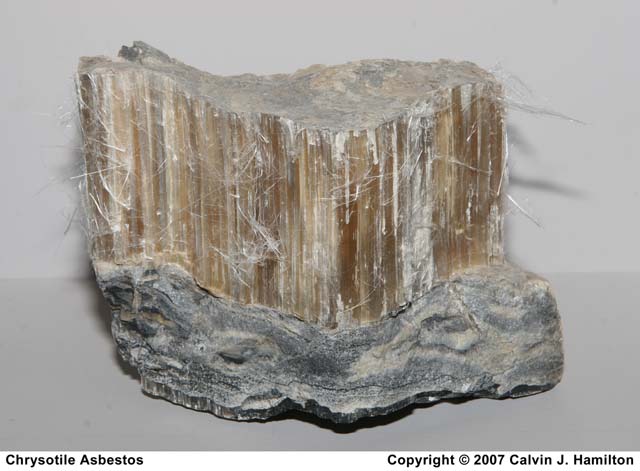This image features a sample of chrysotile asbestos, captured in a detailed photograph credited to Calvin J. Hamilton, Copyright 2007. The mineral sits against a plain gray background, possibly on a table, with a noticeable shadow cast behind it. The lower portion of the mineral exhibits a dark gray, rocky texture, while the upper part transitions into a brown, fibrous formation. Vertical brown and white stripes mark the top section, with thin white fibers extending outward, giving it a somewhat fuzzy appearance. The stark contrast between the rocky base and the fibrous crown, along with the delicate vertical and horizontal patterning, highlights the complexity and texture of the chrysotile asbestos sample.